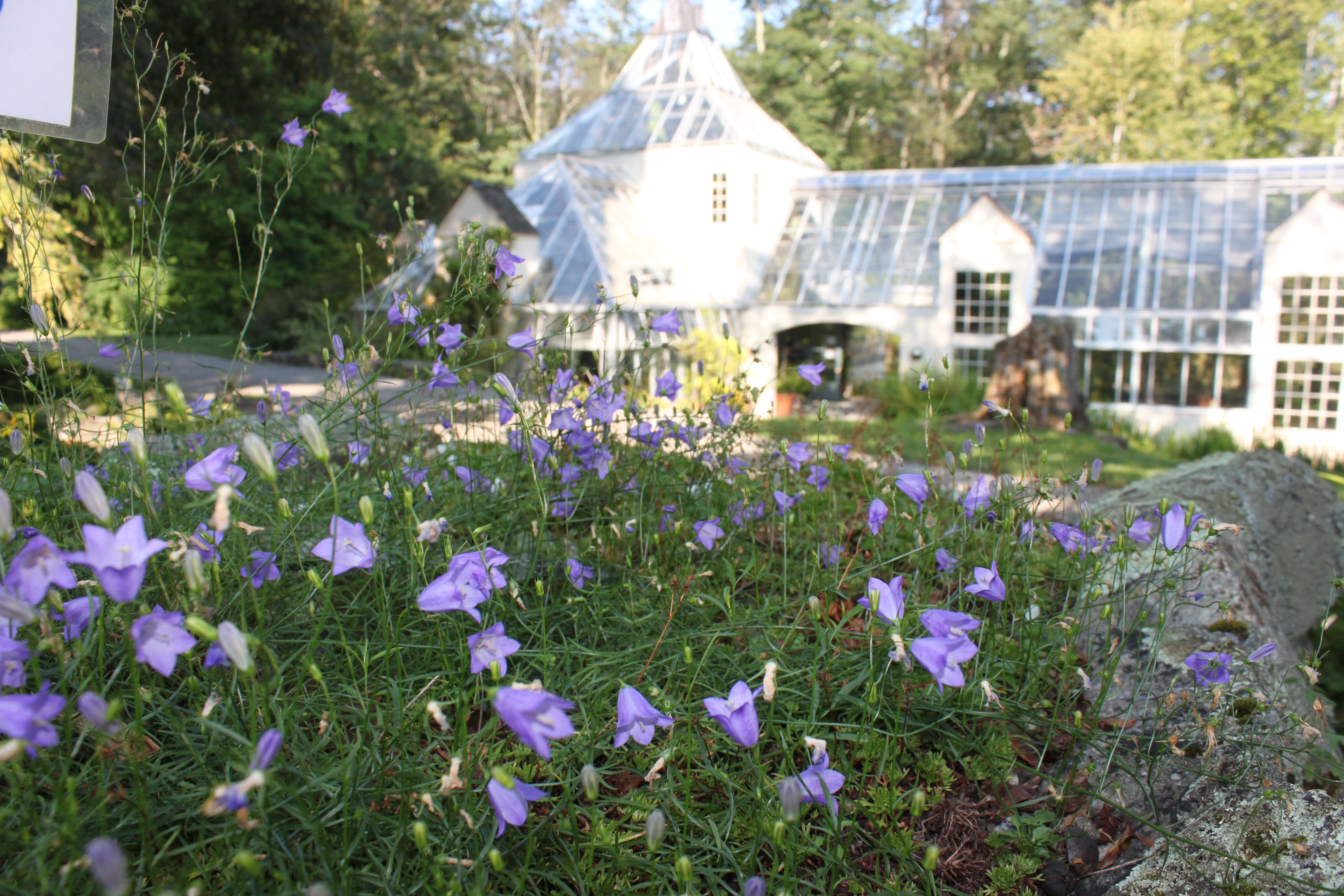In the foreground of this image, there is a lush display of delicate blue and purple, bell-shaped flowers, resembling bluebells, surrounded by abundant ferny greenery. These flowers stretch back to about halfway in the photo, growing beside a rock border, and are spread across a weed and grass patch. Behind this floral foreground, a cement sidewalk or gravel walkway leads the eye towards a striking greenhouse. This elegant conservatory-type structure, featuring a mixture of glass and metal, displays a large entryway at the center, arched windows, and a distinctive domed top on the left side that extends horizontally to the right. The greenhouse, with its transparent roof panels, allows ample sunlight to nurture the plants inside. The background is adorned with tall trees and various green shrubs, creating a serene, verdant atmosphere that frames the entire scene. The image captures a peaceful outdoor setting devoid of people, focusing solely on the natural beauty and architectural interest present.